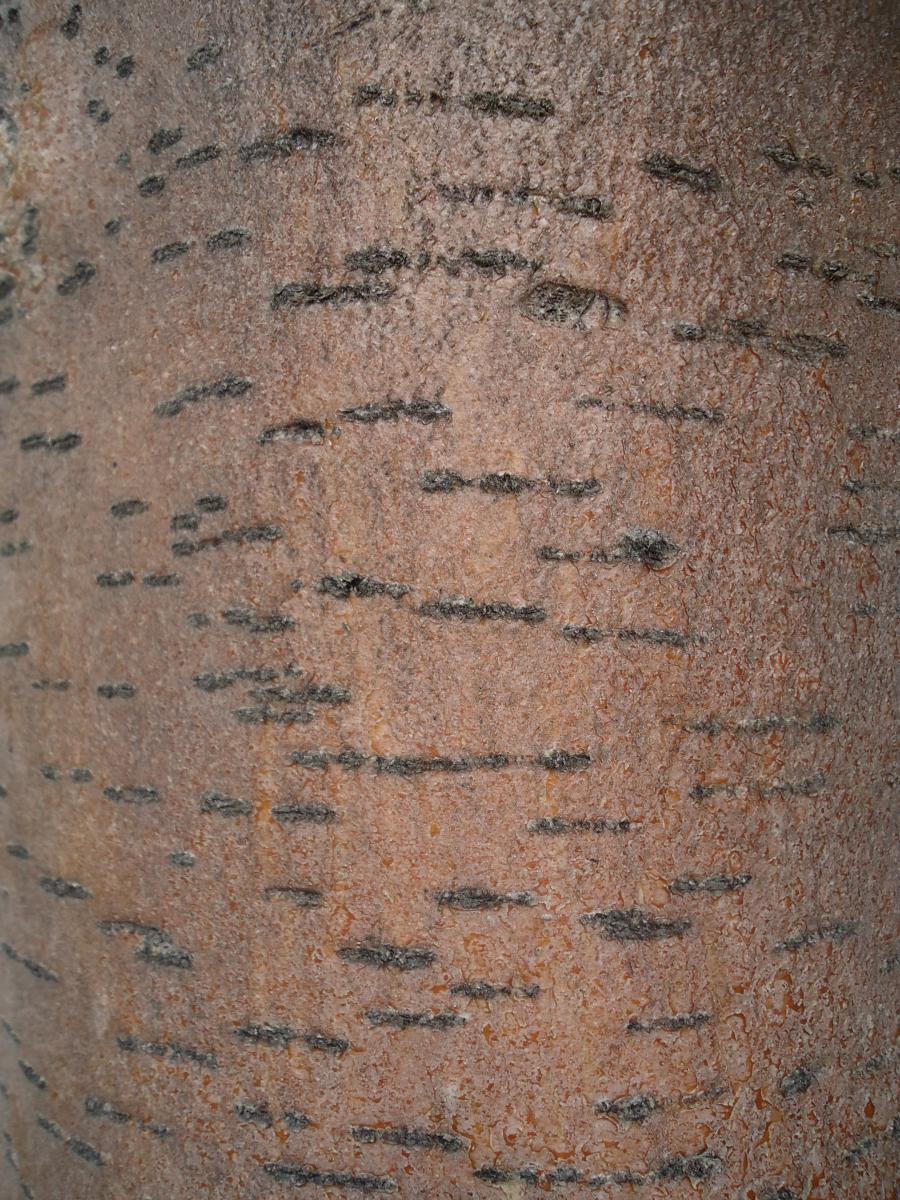The image is a detailed, extreme close-up of a texture that predominantly looks like an orangish-brown tree trunk with a mottled appearance, potentially confused with rock due to its complexity. The surface is covered with irregular, dark gray to black, raised lines that resemble scars or scabs, reminiscent of cat scratches. These lines run vertically from top to bottom, with a more concentrated pattern near the top of the image. The background is filled with grooves and dips, giving the texture an intricate, uneven appearance. The overall effect is one of a smooth yet rugged surface, marked by these crisscrossing lines that create a striking visual pattern across the entire horizontal rectangular image.